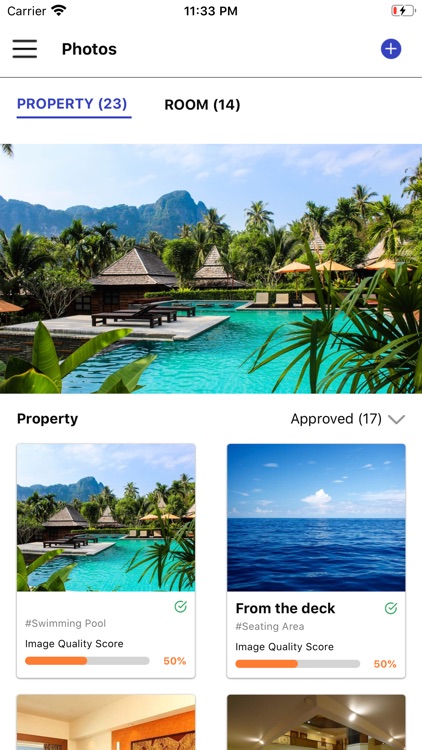**Detailed Caption:**

The image depicts a vacation property featuring several individual cabins, each resembling small, standalone rooms. The primary focus is a large, inviting swimming pool with a striking turquoise hue situated in the center of the property. Surrounding the pool are various seating areas, offering comfortable spots for relaxation. 

The scene is adorned with a variety of colors including turquoise, blue, orange, gray, black, white, green, brown, and off-white. Each cabin and seating area is meticulously designed, contributing to the overall aesthetic appeal of the property. 

The top of the image shows a status bar with data reception symbols and the timestamp "11:33 PM." The battery indicator reveals that the battery is running low. Text annotations around the image include labels such as "Photos Property 23 Room 14" and hashtags like "#swimmingpool" indicating the main feature. Image quality scores are noted as 50%, with the mention of 17 approved entries from the deck and the inclusion of "#seatingarea".

Though only the upper portion of the image is visible, three distinct photos can be identified – one of which repeats. The background of the annotations is primarily white with black fonts, contributing to a clean and minimalist overlay.